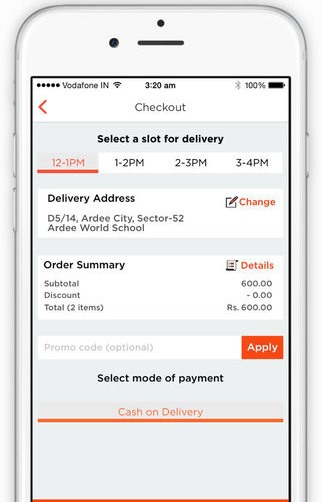The image showcases a white smartphone displaying a checkout screen on the Vodafone app. The screen is set against a white and gray background adorned with red lines and various pieces of black text. At the top of the screen, it reads "Vodafone IN," followed by "3:20 AM," and indicates that the phone is "100% charged." 

There is a red arrow pointing left next to the text "Checkout," guiding the user through the process. Further down, there is a section titled "Select a slot for delivery," with the currently selected slot being "12-1 PM." Other available time slots are "1-2 PM," "2-3 PM," and "3-4 PM."

Below this, the delivery address is displayed, accompanied by an option to change it by clicking on the red "Change" text. The order summary informs the user of a total cost of $600 for two items, with no discounts applied. The word "Details" is highlighted in red, presumably linking to more detailed information about the order.

A rectangular box for entering a promo code, labeled as optional, is positioned next, along with an "Apply" button. The selected mode of payment is "Cash on Delivery." At the very bottom of the screen, two red horizontal lines span the width of the phone’s display, closing off the checkout section.